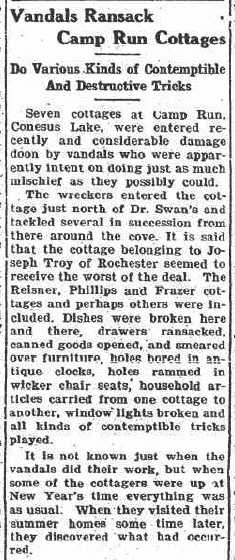The black-and-white newspaper article, rectangular in shape, is titled "Vandals Ransack Camp Run Cottages" with a subtitle "Do Various Kinds of Contemptible and Destructive Tricks." According to the article, seven cottages at Camp Run, Concius Lake, were recently targeted by vandals intent on causing extensive mischief. The vandals began their spree at the cottage just north of Dr. Swann's and continued their destruction around the cove. Among the affected properties, the one belonging to Joseph Troy of Rochester suffered the worst damage. Other cottages mentioned include those of Reisner, Phillips, and Frazier. The destruction was extensive: dishes were broken, drawers ransacked, canned goods opened and smeared over furniture, holes bored in antique clocks, and seats of wicker chairs were vandalized. Household items were moved from one cottage to another, windows were broken, and numerous contemptible tricks were played. The exact time of the vandalism is unknown, but it was noted that everything was normal during a visit at New Year's, with the damage discovered only upon later inspection.